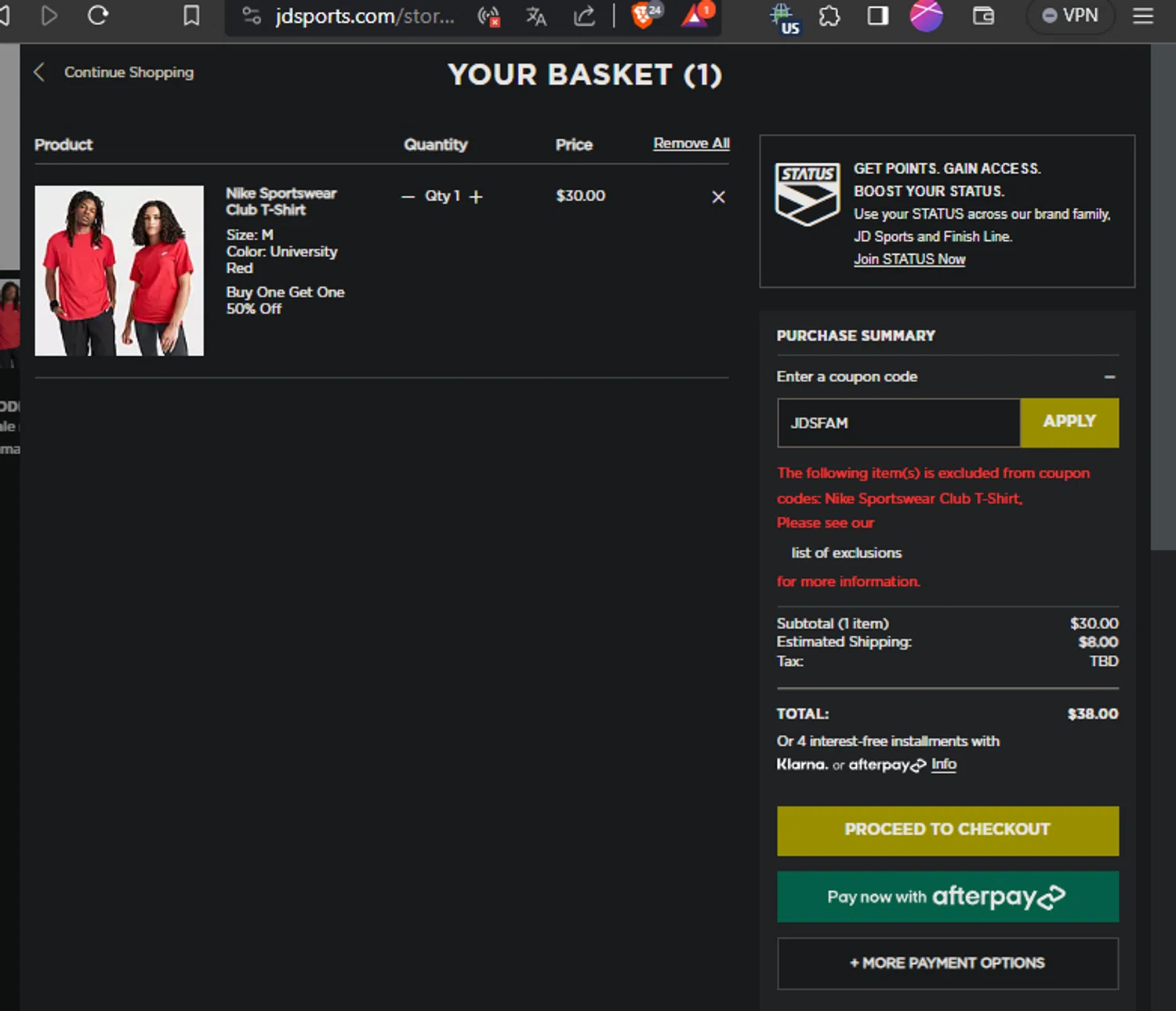This image is a detailed screenshot from the online retailer JD Sports, showcasing the shopping cart page against a black background. At the top, the browser window reveals part of the web address, "jdsports.com/...".

The page prominently displays the heading "Your Basket (1)" in white text, indicating one item in the cart. The product photo features two models: a Black man with long dreadlocks and a white woman with shoulder-length dark brown hair; both are dressed in matching red Nike Sportswear Club t-shirts and black pants against a white backdrop.

Next to the image, the product details are clearly listed: "Nike Sportswear Club T-shirt, Size M, Color University Red," along with a promotional offer: "Buy One Get One 50% Off." The price of the t-shirt is marked as $30.

On the right side of the page, there's a section to apply a coupon code, which appears to have already been used. Below this, some red text appears, though it's difficult to read. The subtotal is stated in white text as $30, with estimated shipping costs of $8 and taxes yet to be determined (TBD). The total amount is shown as $38.

Further down, there's an option for "4 interest-free installments with Klarna or Afterpay." Below this, a greenish-gold button labeled "Proceed to Checkout" in white text stands out, followed by a green button for "Pay Now with Afterpay" and a black button for "More Payment Options."